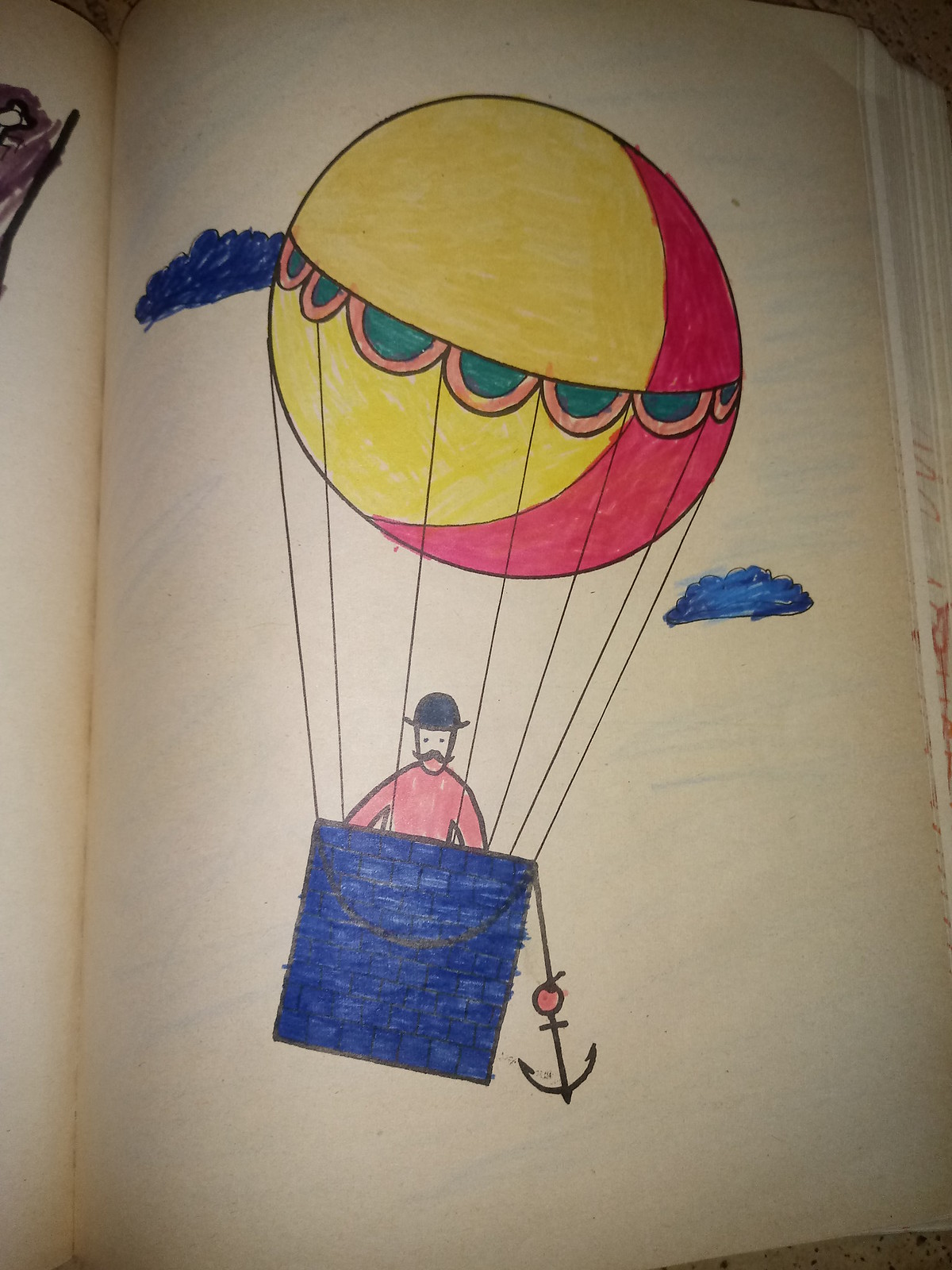The photograph captures an open page from a coloring book that has been meticulously filled in. The image depicts a man in a hot air balloon, which is spherical and adorned with doilies in the center. The balloon has been primarily colored yellow with markers, featuring a crescent-shaped red highlight prominently on the lower right side, along with green and red patterned drapings around its middle. The man inside the balloon, who looks like he's from the turn of the century with a fancy mustache, wears a blue bowler hat and a red (or possibly pink) long-sleeve shirt. The basket of the hot air balloon is colored blue and has an anchor hanging off its side, giving the impression of it tipping slightly. Surrounding the balloon are dark blue clouds that match the color of the basket, set against a light blue background. In the upper left corner of the photograph, part of another page from the coloring book peeks through, showing some black and brown scribbles, suggesting other completed illustrations.